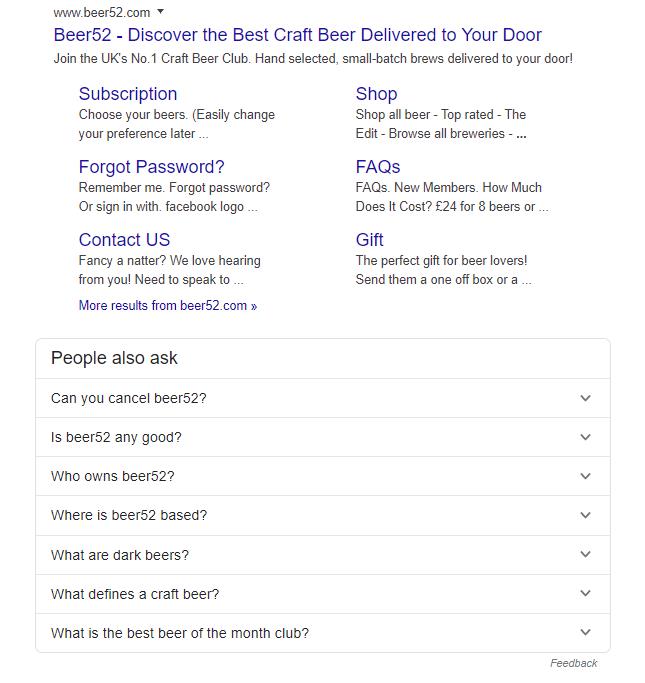The image depicts a search result screen from Google. In the top left corner, the URL "www.beer52.com" is displayed with a down arrow next to it. Directly below, the search result title "Beer 52 – Hype it, discover the best craft beer delivered to your door" is shown in the typical blue font used in search results, followed by a brief sentence in black font describing the service. 

Below this, the screen is divided into two columns, each containing three clickable options in blue font. The left column includes "Subscription," "Forgot Password," and "Contact Us," while the right column features "Shop," "FAQs," and "Gift." Each of these options has a succinct one-sentence description beneath it. Notably, under the "Contact Us" option, there is an additional link labeled "More results from beer52.com" in blue font.

Further down, the screen displays a table-like structure with seven rows. The first row serves as a heading, bolded in black font, reading "People also ask." This is followed by six questions in regular black font, including "Can you cancel Beer 52?", "Is Beer 52 any good?", and "What is the best beer of the month club?" Each question has a down arrow to its right, indicating expandable content for more information.

In the lower right-hand corner, the word "Feedback" is visible, suggesting an option for user feedback on the search results.

This detailed layout provides a clear vision of the search result page and its various navigational elements related to Beer 52.